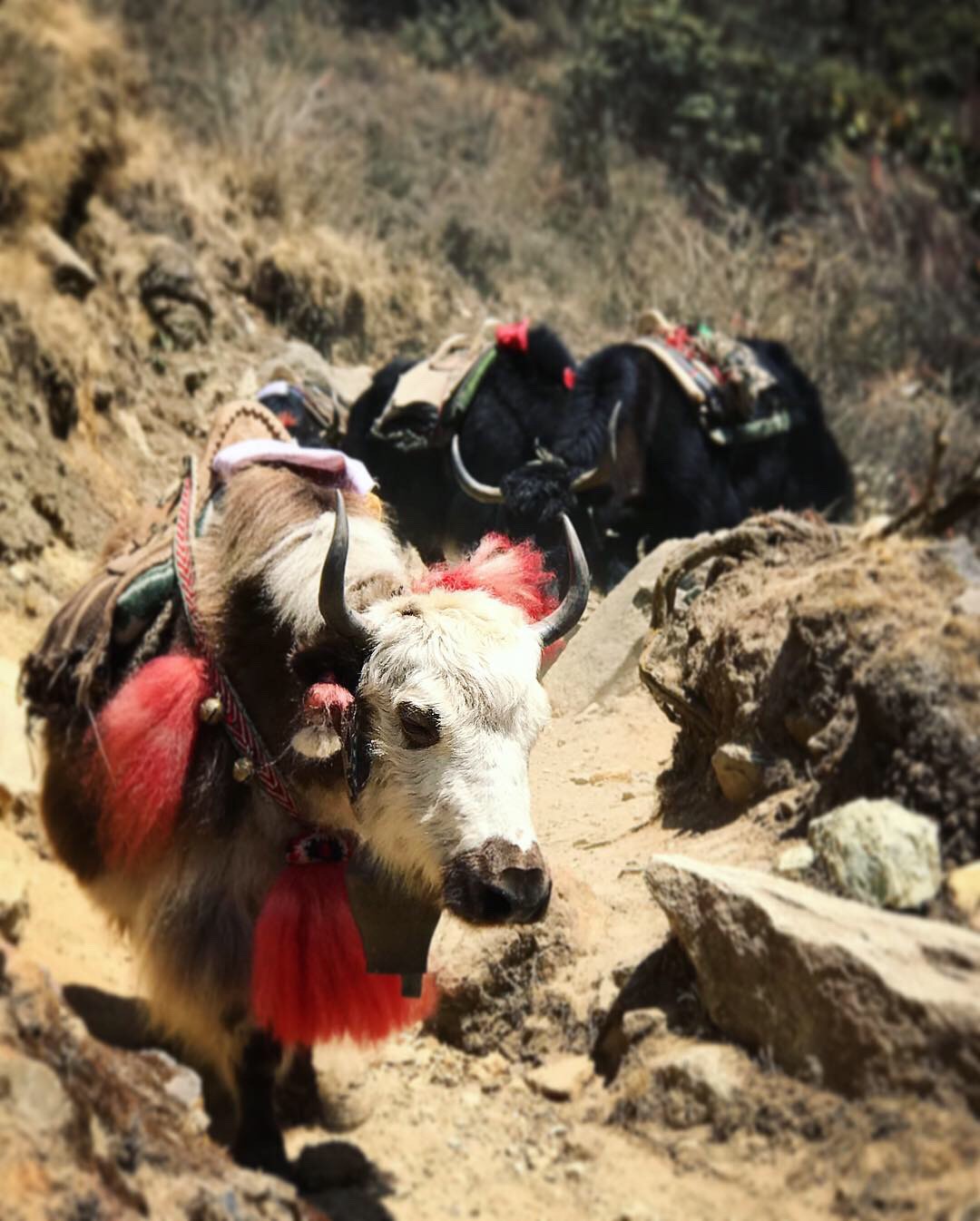In a dry, rugged landscape, under the bright sun, three animals traverse a rocky path flanked by scrubby vegetation and large boulders. The foreground features a distinct black and white animal, presumably a domesticated yak, adorned with vibrant red feathers, a riding saddle, and a blanket. It has a white face and strikingly sharp, curved horns. Behind it, two completely black animals, likely domesticated rams, follow, each with curved horns and packs decorated in red and green. The rocky terrain is unyielding, and the sparse greenery and brown, dried-out bushes underscore the arid environment. The photograph, evocative of an older era, captures a moment of hardy perseverance amidst the harsh landscape.